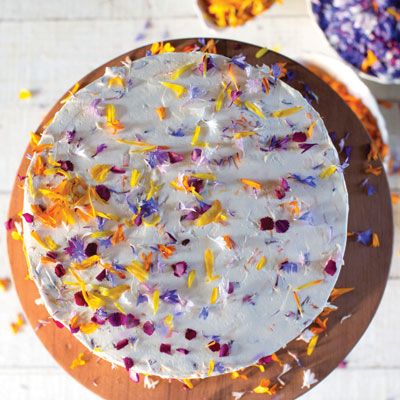The image depicts a round cake placed on a raised wooden cake stand, viewed from a top-down perspective. The cake is smoothly frosted in a light blue color and is adorned with an assortment of decorative elements resembling flower petals in various shades of yellow, purple, and white. These colorful flecks are scattered across the cake's frosting, with some spilling over onto the wooden stand and the white surface that lies underneath. Additionally, in the background, there are three bowls, each containing a different color of the decorative sprinkles—likely the same yellow, purple, and white seen on the cake. The entire scene is set against a white wooden tabletop, creating a visually appealing contrast between the vibrant cake and its minimalist surroundings.